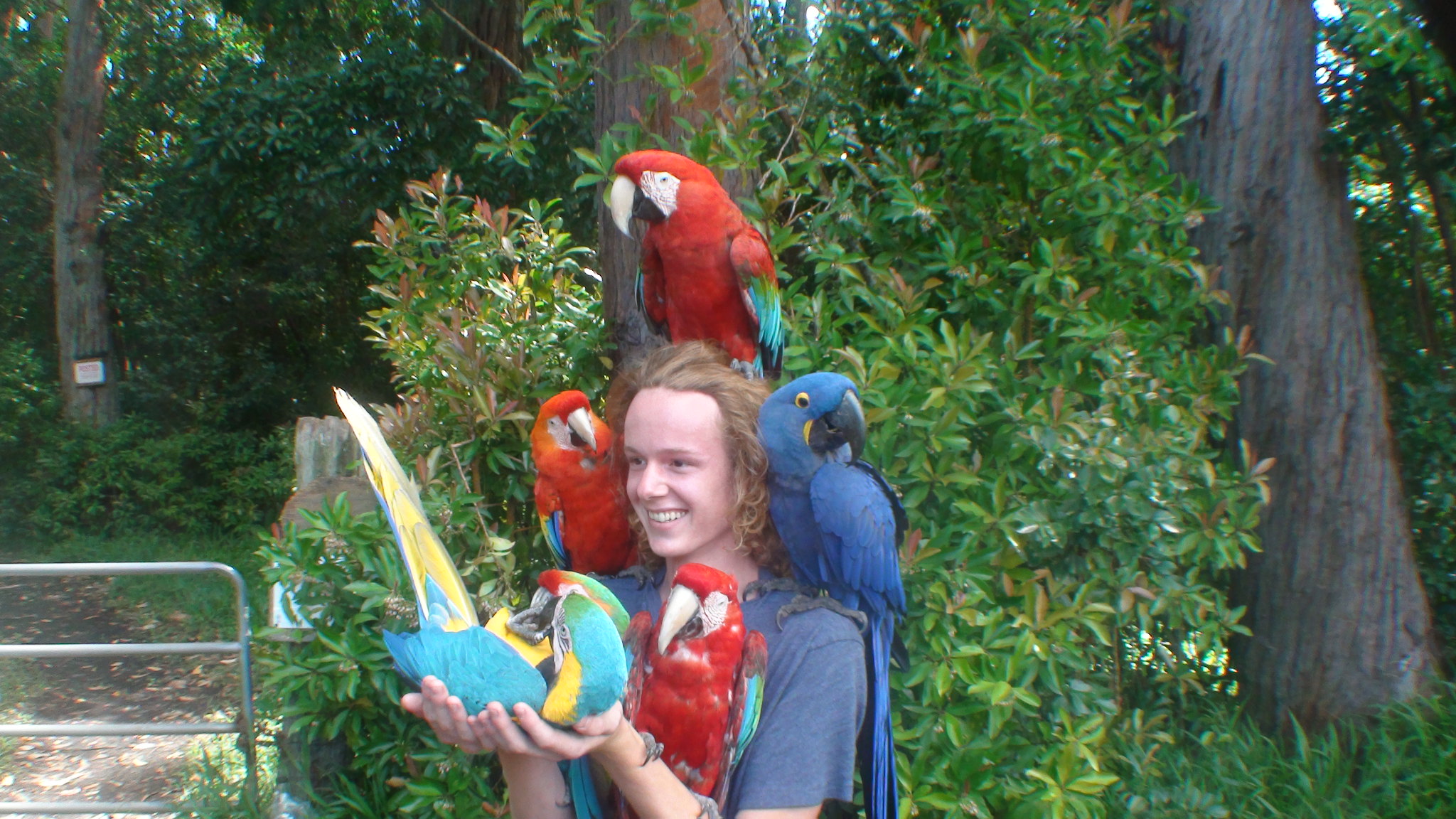This color photograph captures a young man, likely a tourist, enjoying a day out at what appears to be a zoo or animal sanctuary surrounded by lush greenery and tall trees. The man with long, slightly gingerish curly hair is facing slightly to the left, smiling and looking out of the frame. He is wearing a blue t-shirt and holding his arms upwards at a 45-degree angle with his hands cupped. Perched all around him are five vibrant parrots in various striking hues: a turquoise parrot with a yellow tail in his cupped hands, a parrot with red and turquoise feathers gripping his forearm, one parrot on each of his shoulders, and another parrot sitting on top of his head. The background features abundant green foliage, a large diagonal tree trunk on the right, and a maple railing with three horizontal rails on the left side of the frame.